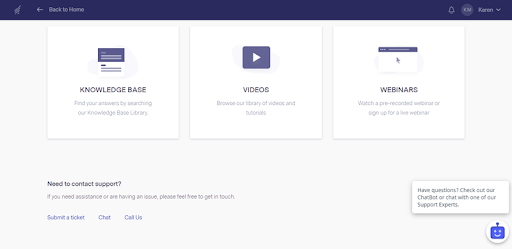Sure, here is a cleaned-up and detailed caption for the image described:

---

The screen displays a navigation bar across the top, featuring a dark navy blue background. On the far left, there is a white left-pointing arrow accompanied by the text "Back to Home." On the far right, there is a bell icon next to a circle labeled "Karen," which seems to offer a drop-down menu. 

Below the navigation bar, three white boxes are aligned in a row. The first box on the left is labeled "Knowledge Base" with the subtext, "Find your answers by searching our knowledge base." The middle box, titled "Videos," invites users to "Browse our library of videos." The last box on the right states "Webinars" and encourages users to "Watch pre-recorded webinars or sign up for a live webinar." The image appears to have very poor resolution, making the text somewhat difficult to read.

Further down, the left section of the screen has a heading, "Need to Contact Support?" followed by the text, "If you need assistance or are having an issue, please feel free to get in touch." Beneath this, there are three blue clickable links labeled "Submit a Ticket," "Chat," and "Call Us."

To the right, there is a section titled "Have a Question?" which prompts users to "Check out our chat bot or chat with one of our support experts." This section is accompanied by a blue chat bot icon.

---